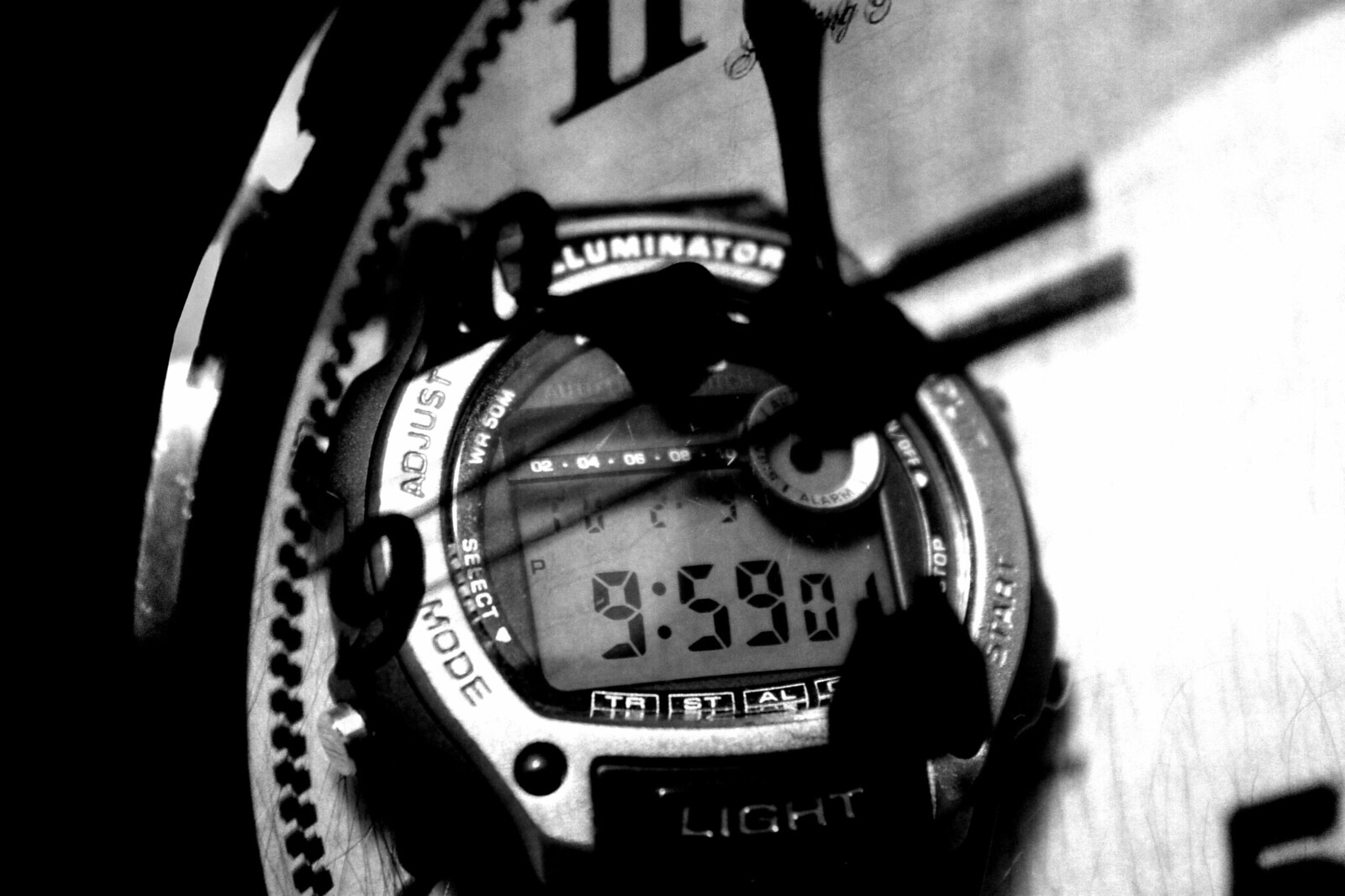This highly detailed black and white photograph offers an extremely zoomed-in view of a pocket watch, which forms the focal point of the image. The pocket watch is prominently positioned towards the center-left of the frame, displaying intricate details with striking clarity. At the very bottom of the image, the top part of the numeral "5" is visible in bold black. Above this number, a series of white streaks of light create a contrast against the dark backdrop.

The pocket watch itself features a silver ring encircling its face, adding an elegant touch to its design. Positioned at the bottom of the watch face is a black rectangle that bears the inscription "Light." The time displayed on the watch is precisely 9:59, with an additional zero appearing at the end of the numerals, which are in black. Two arrows are seen crossing diagonally over the top of the pocket watch, adding a sense of dynamism to the scene.

In the background, a faint image of a gray clock face can be discerned, adding another layer of depth and complexity to the composition. A single silver line runs vertically along the left-hand side of the image, contrasting sharply with the otherwise solid black background. The overall monochromatic scheme enhances the timeless feel of the photograph, drawing attention to the fine details and textures of the pocket watch.